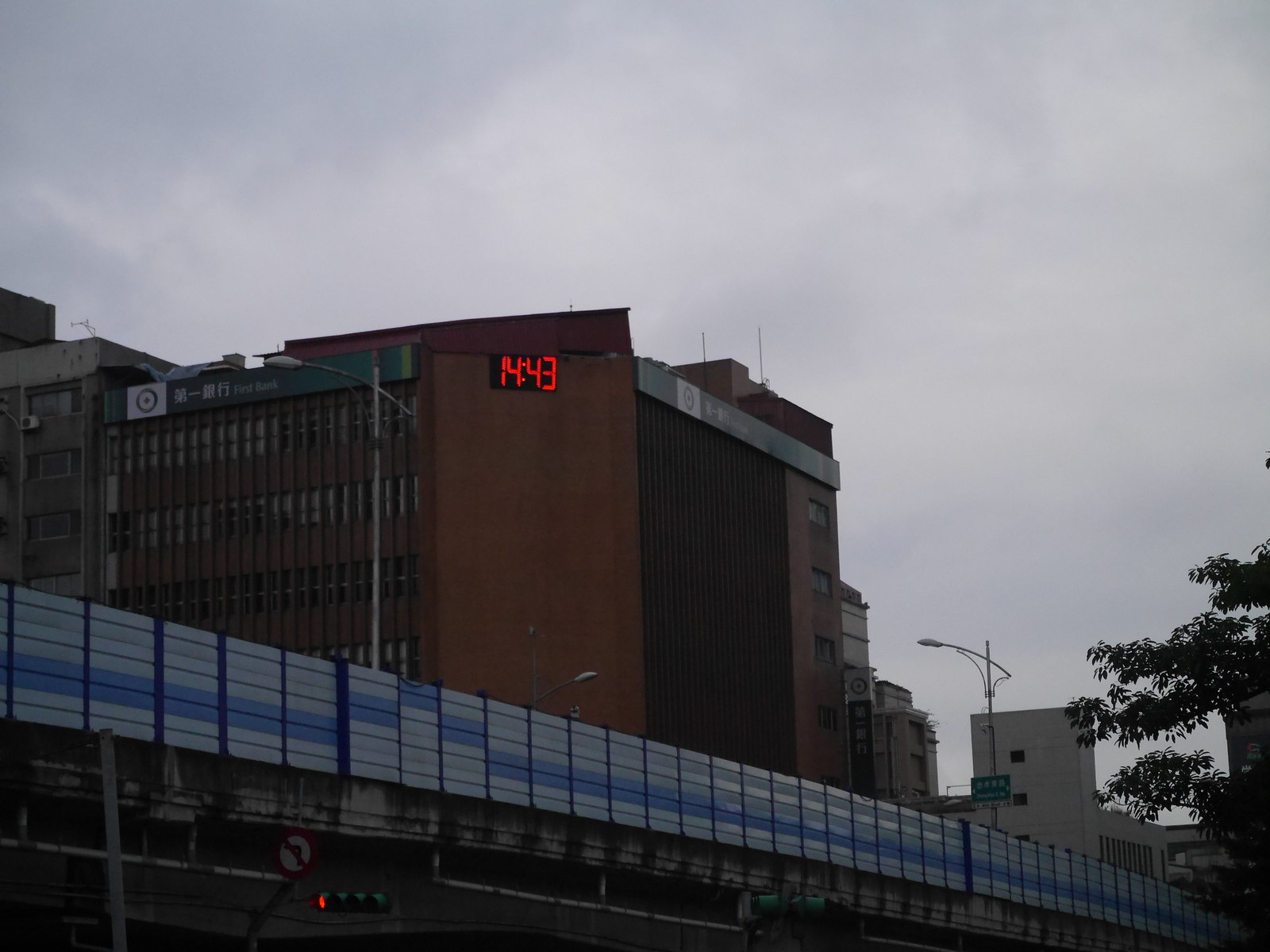The image captures a bustling metropolitan area with distinct architectural and infrastructural features. In the foreground, there's a modern train bridge adorned with an aesthetically pleasing fence, featuring blue, black, and white stripes. This bridge adds a contemporary touch to the urban landscape. Just behind the bridge stands a large brick building, crafted from either red or brown brick, boasting a modern design. Tall vertical lines accentuate the building's facade, highlighting its numerous windows. A black horizontal sign stretches across the top of the building, though its inscription is unreadable; it likely denotes the name of the company or the building itself. A prominent digital clock with red numerals displaying "14:43" in military time is mounted on the building's side.

Further in the background, another gray building with a more aged appearance peeks over, contrasting with the modern structures in the foreground. Additional buildings fade into the distance, appearing less contemporary and detailed. One discernible building features an analog clock on its facade.

Several lamp posts line the train bridge, contributing to the urban infrastructure, and a green traffic sign is attached to one of the posts. Below the bridge, traffic lights are visible along with a "No Left Turn" sign, although the road itself is out of view. The scene is set on a cloudy day, with a gray, misty sky casting a subdued light over the cityscape. A small tree is visible on the left side of the frame, adding a touch of greenery to the urban environment.